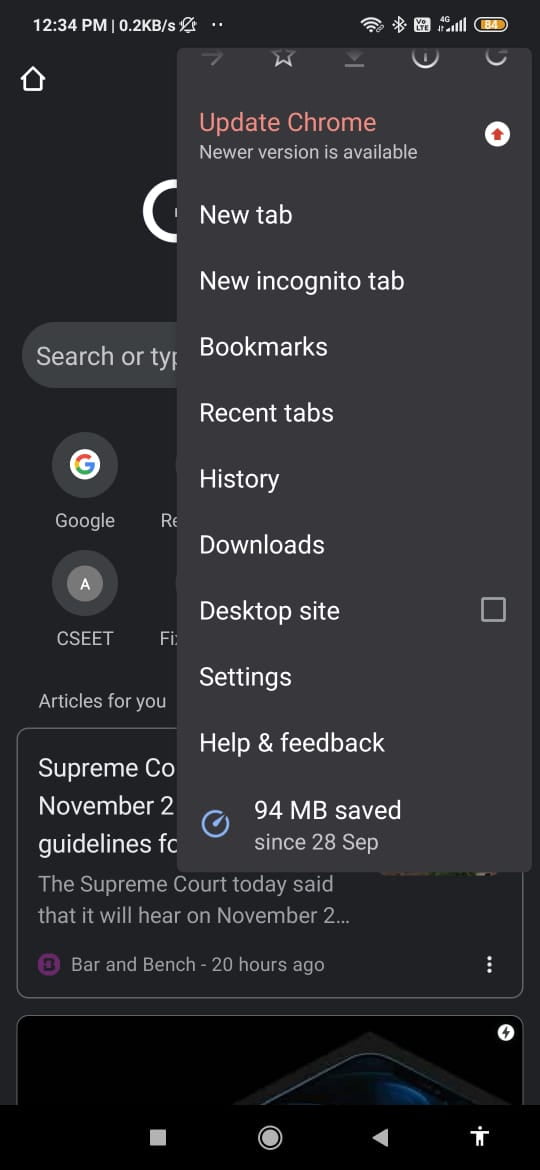At a first glance, the image appears to be a screenshot of a smartphone's screen. The screenshot shows a cell phone interface with a black background. The time displayed on the phone is 12:34 p.m. on the top-left corner. Just below the time, it indicates a network speed of 0.2 kb per second, and there is no alarm icon present. The battery is at 84% charge.

From the right side of the screen, a menu tab is visible. This tab lists several options: "New incognito tab," "Bookmarks," "Recent tabs," "History," "Downloads," "Desktop site," "Settings," and "Help and feedback." Beside the "Desktop site" option, there is an unchecked square box. The menu also mentions "94MB saved since 28 September."

In the background, partially obscured by the menu, the Google Chrome app is open. At the top, there is a text box with the words "search or type" inside it, indicating the search bar. Below the search bar, the Google logo is visible alongside another logo featuring a seated figure with the letter "A" in it.

Below the logos, a news headline reads: "Supreme Court November guidelines." Following this, there is a brief description: "The Supreme Court today said that it will hear on November 2..." This particular article appears to be from "bar and bench," dated 20 hours ago.

Additionally, in the upper-right corner, there is a red alert prompting the user to update Google Chrome, indicating that a newer version is available. The alert emphasizes the importance of updating the browser.

Overall, the screenshot displays a typical smartphone interface showing various statuses and notifications, alongside a user interacting with the Google Chrome app's settings menu.